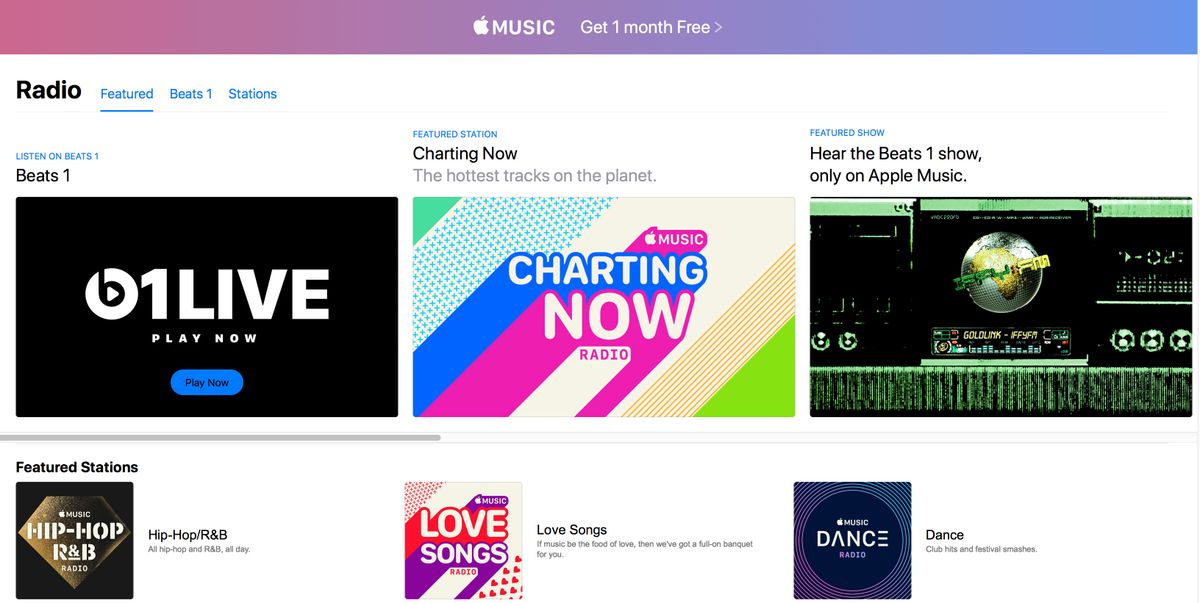The image is a screenshot of the Apple Music website. At the top, there is a slim, gradient banner that transitions from pink on the left to a light blue on the right, creating a purple hue in the middle. In the center of this banner, the Apple logo and the word "MUSIC" are prominently displayed in white text, accompanied by the offer, "Get one month free."

Beneath the banner is a header titled "Radio," with three tabs positioned to its right: "Featured" (which is currently selected), "Beats 1," and "Stations." Below this header, three large thumbnail images are displayed, each with titles and descriptions.

- The first thumbnail on the left features a black background with "1LIVE" in bold white letters accompanied by "Beats 1" at the top.
- The central thumbnail is vibrant, featuring diagonal stripes in green, blue, hot pink, and beige. The text in the center, "Charting Now," is written in blue and hot pink, with "Apple Music," "Radio," and "Featured Station" labels. The accompanying description reads, "Charting Now: the hottest tracks on the planet."
- The thumbnail on the right displays a green and black image with indistinct text and is labeled "Featured Show" above, with the description, "hear the Beats 1 show only on Apple Music."

At the very bottom of the image, three smaller thumbnail images represent "Featured Stations": "Hip Hop and R&B," "Love Songs," and "Dance."